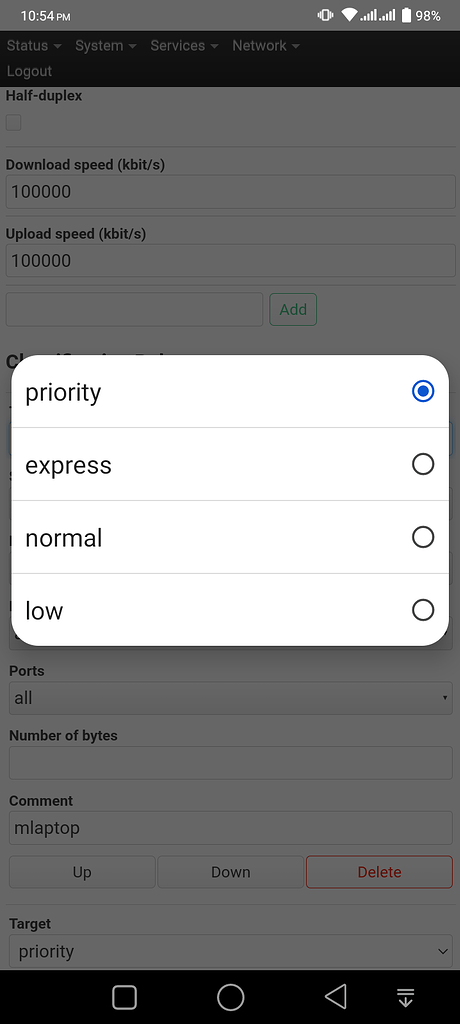In this image, the backdrop is a dark gray background. At the very top, the time is displayed as "10:54 PM," alongside a battery icon indicating a 98% charge. Below this, there is a blue rectangular block containing some text.

Continuing, the dark gray area prominently displays "Half Duplex Download Speed" and "Upload Speed." In the center of the image, there is a white box labeled "Priority." This box features a blue circle with another blue circle inside it, situated above a horizontal line. Beneath this, there are three options for priority settings: "Express," "Normal," and "Low," each accompanied by an empty circle that likely serves as selection indicators.

The dark gray section also contains the labels "Ports," "Number of Bytes," "Comment," and "Laptop." Adjacent to these, there are up and down arrow buttons alongside a delete button. Furthermore, within this gray area, there are labels for "Target" and "Priority."

At the bottom of the image, there is a black bar containing the usual navigation icons: a square, a circle, and a triangle, with two horizontal lines above them suggesting a status bar.